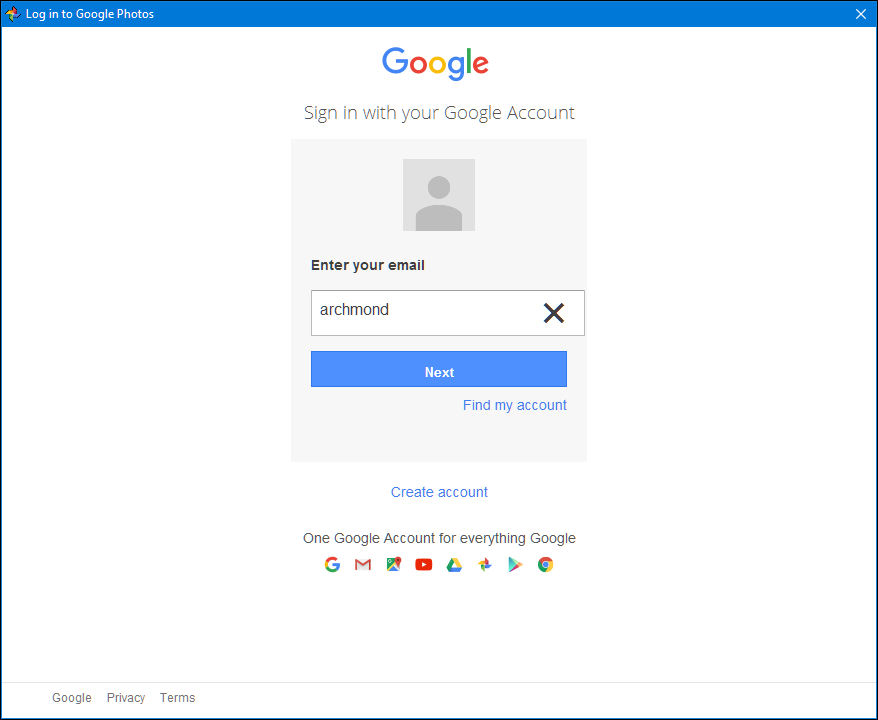A screenshot of an older Google sign-in page appears on what seems to be a Windows XP or a Windows 7 system customized to resemble Windows XP. The interface strongly suggests it is from the early to mid-2010s. The window displays a Google Photos application, distinct from the web-based version. At the top, it features the classic Google logo, followed by a prompt to "Sign in with your Google Account." Below, there's a field where a user has typed in "Archmond" (A-R-C-H-M-O-N-D) as their email. Options such as "Next," "Find my account," and "Create account" are available for navigation.

A tagline beneath states, "One Google Account for everything Google," accompanied by a single 'G' Google logo, and icons for Google Mail, Google Maps, YouTube, Google Drive, Google Photos, Play Store, and Google Chrome. The bottom left corner includes links to "Google Privacy" and "Terms." The profile picture placeholder is a square, in contrast to the round images Google uses currently. Additionally, the outdated Google Play Store logo displays a blue triangle with overlapped yellow and red edges, reinforcing the timestamp of this version being two iterations old.